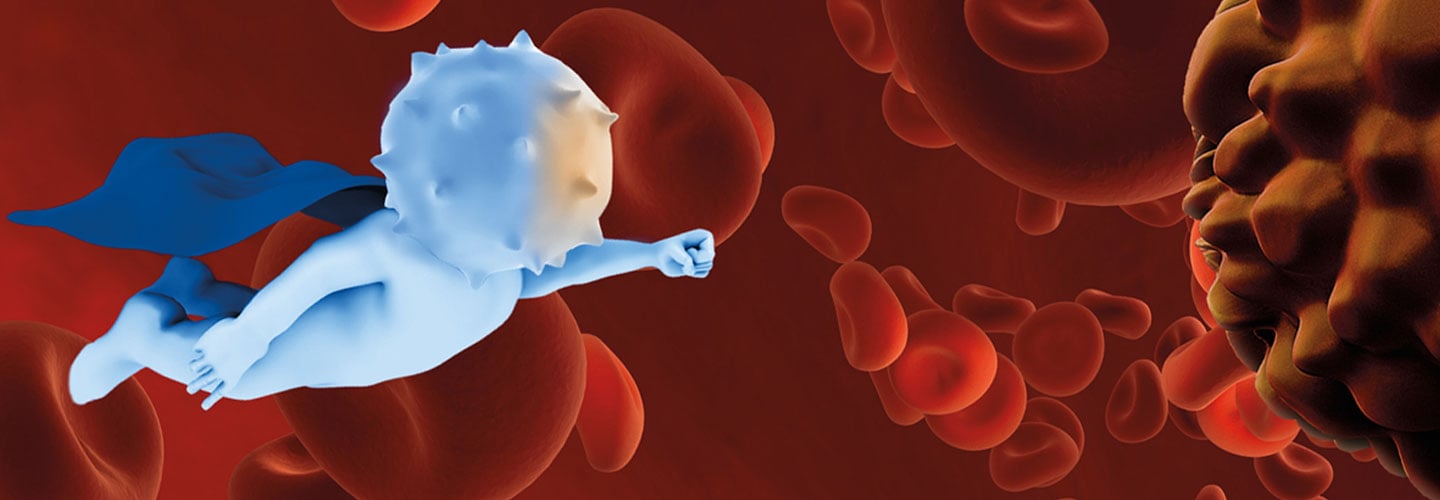In this detailed digital rendering, we see an animated scene that might be intended for a biology lesson. The backdrop is a vibrant red, resembling a sky filled with red blood cells, some of which are depicted as little round dots or amoebas floating around. A prominent feature on the right side is a brownish, textured pattern that appears similar to a pine cone or a spiky, unhealthy cell. 

In contrast, a striking figure takes center stage, depicted as a light blue, angelic character flying with a darker blue cape reminiscent of a superhero. This figure, resembling a Cupid or an animated cell with finger-like extensions, soars with its left hand extended forward and its right hand trailing behind, emulating a Superman-like pose. Notably, its face is an unusual circular form with protruding lines or spheres, adding a quirky, almost bizarre element to the scene. The blue-caped figure appears to be in motion towards the brown, spiky object on the right, evoking a sense of action and purpose in this surreal, educational depiction.